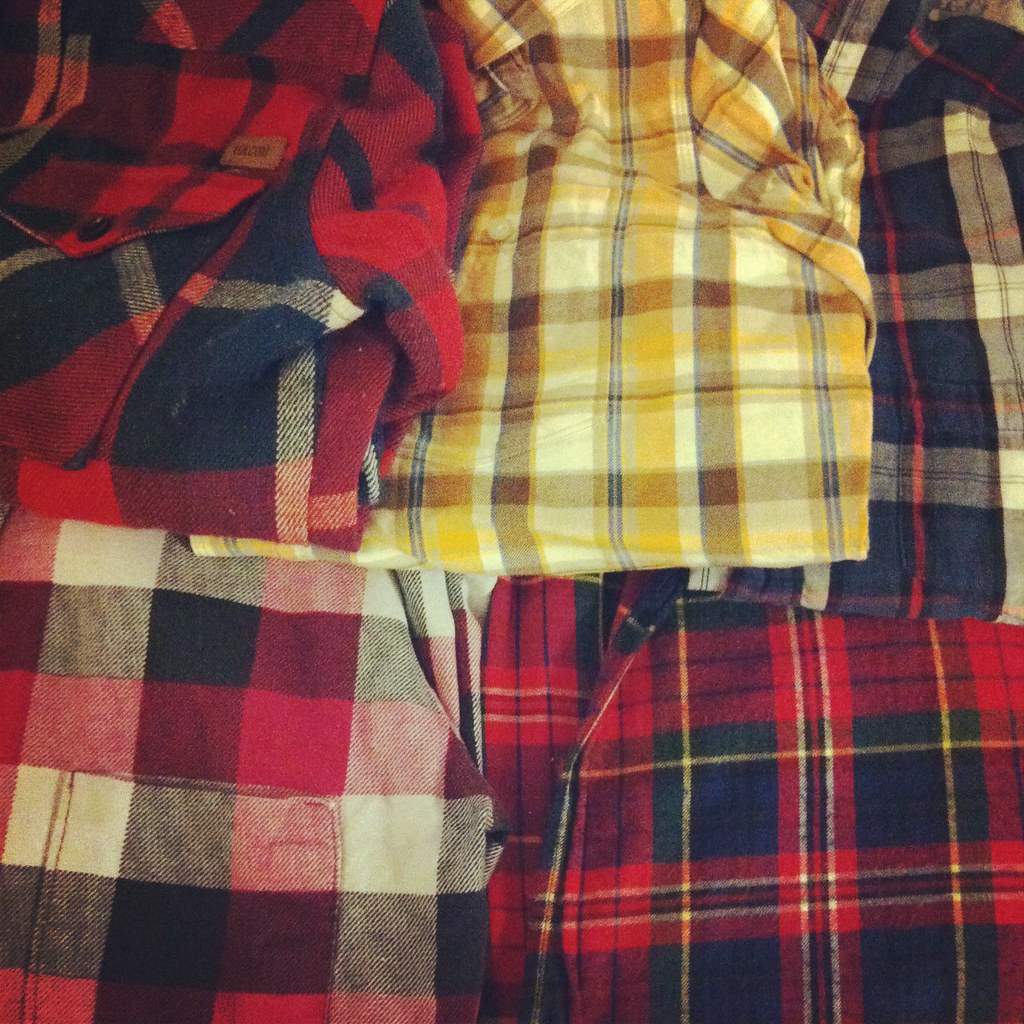This image showcases a collection of five distinctively patterned flannel shirts, all meticulously folded to occupy the entire frame. In the upper left corner is a red and blue tartan flannel shirt, featuring a pocket with a dark navy blue button and a small, illegible label. Next to it, in the upper middle, is a yellow, brown, and blue striped flannel shirt. Moving to the upper right, there is a predominantly blue and white plaid shirt with red and grey accents. Below this, to the left, lies a more block-patterned flannel with maroon, pink, grey, and white squares, displaying another pocket. Finally, in the far bottom right, a flannel shirt showcases a vibrant mix of red, green, blue, black, and white, evoking a traditional and festive Christmas feel.